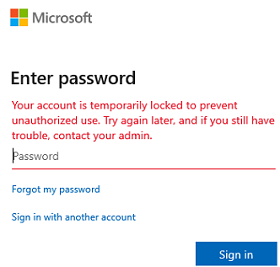The screenshot is displayed against a solid white background. In the upper left corner, the word "Microsoft" is written in gray. To the left of this text is the Microsoft logo, which consists of four small squares arranged to form a larger square. The color arrangement of the squares is as follows: the top left square is red, the top right square is green, the bottom right square is yellow, and the bottom left square is blue.

Below the logo, there is a prominent, bold heading in large black text that reads "Enter password." Underneath this heading, there is a cautionary message in smaller red text that states: "Your account is temporarily locked to prevent unauthorized use. Try again later and if you still have trouble contact your admin."

Further down, the mouse cursor is positioned over the gray text that says "password." Below this, in small blue text, are two interactive options: "Forgot my password" and "Sign in with another account."

Finally, in the lower right corner, there is a blue action button labeled "Sign in."